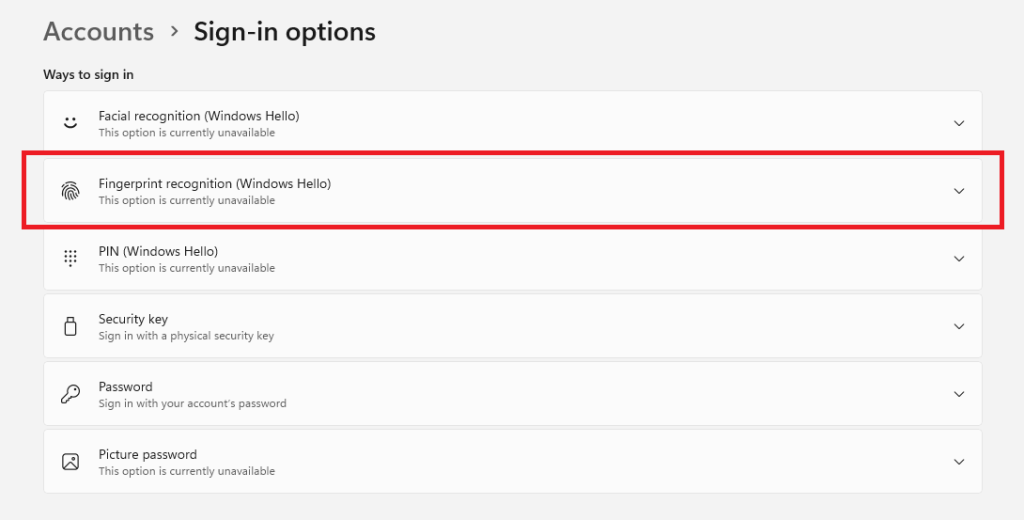The image is a screenshot of a computer screen displaying a user accounts settings menu. The main focus is a horizontal rectangle with a gray border, containing white space in the center with several lines of text and symbols. 

At the top within the gray border, the word "Accounts" is prominently displayed. Below it is an arrow icon followed by the text "Sign-in options," indicating the various available methods for user authentication.

The list of sign-in options, each on a separate line, is as follows:
1. A happy face icon next to the text "Facial recognition (Windows Hello)".
2. A fingerprint icon next to the text "Fingerprint recognition (Windows Hello)".
3. A series of dots icon next to the text "PIN (Windows Hello)".
4. A padlock icon next to the text "Security key".
5. A key icon next to the text "Password".
6. A picture frame icon next to the text "Picture password".

In the image, the line for "Fingerprint recognition (Windows Hello)" is highlighted with a prominent red rectangle, indicating that this option has been selected or clicked on. The red highlighting draws attention to this particular line among the other sign-in options.

This detailed depiction captures the visual and functional elements of the sign-in options page within the user accounts settings on a computer screen.